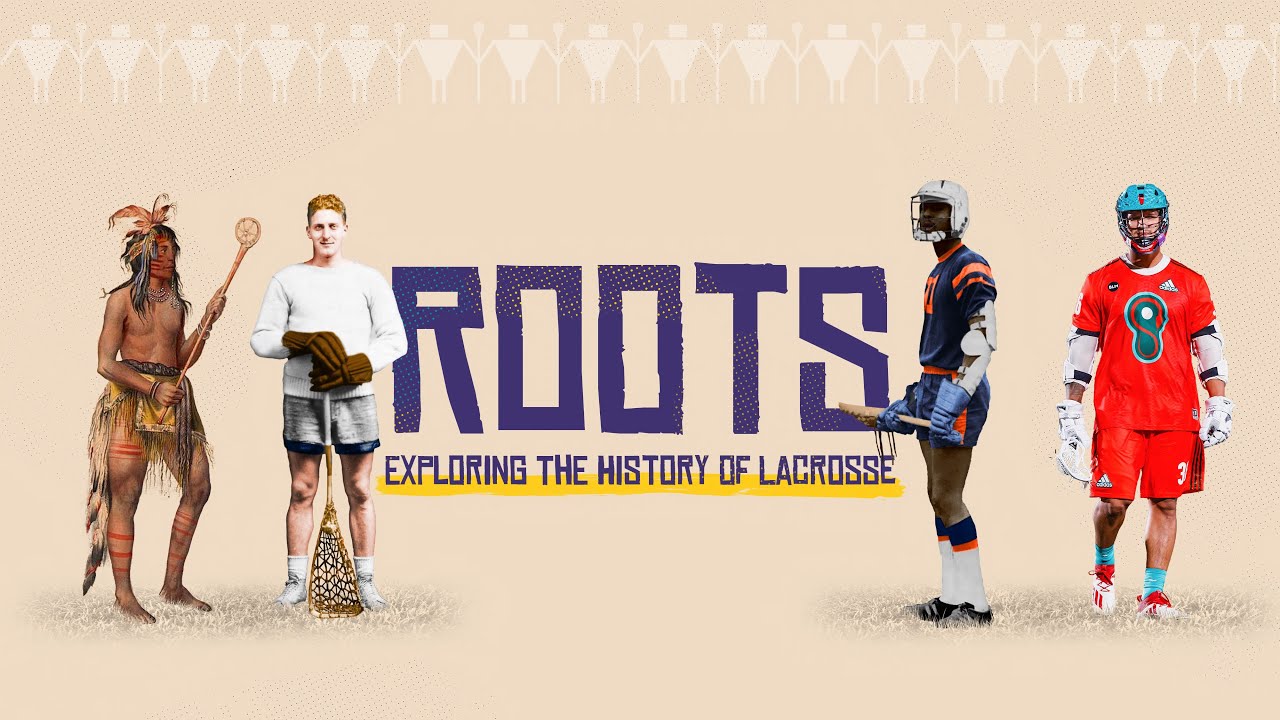The promotional image, which resembles a sepia-toned poster for a documentary or book titled "Roots," vividly captures the evolutionary history of lacrosse. Dominantly displayed in the center are the large, bold purple words "Roots," and beneath, in smaller but still prominent purple text, the subtitle "Exploring the History of Lacrosse," highlighted with a yellow underline. 

The visual narrative is divided into two sections by this central text. On the left, we see a progression starting with a Native American man, shirtless and adorned with traditional feathering in his hair, holding an early, rudimentary lacrosse stick. Beside him stands a white man with reddish-blonde hair, clad in a white shirt and brown gloves, gripping a slightly more advanced lacrosse stick. On the right side, the evolution continues with a black man in a blue and orange jersey, equipped with modern gear and a safety helmet, showcasing a contemporary lacrosse stick. Finally, on the far right, a man fully outfitted in a bright blue safety helmet, red Adidas jersey, matching red shorts, white gloves, and the latest lacrosse stick underscores the modern era of the sport.

The background subtly features a repeating pattern of stick-figure lacrosse players, adding a historical texture to the image, while emphasizing the various stages and cultural significance of lacrosse through the ages.